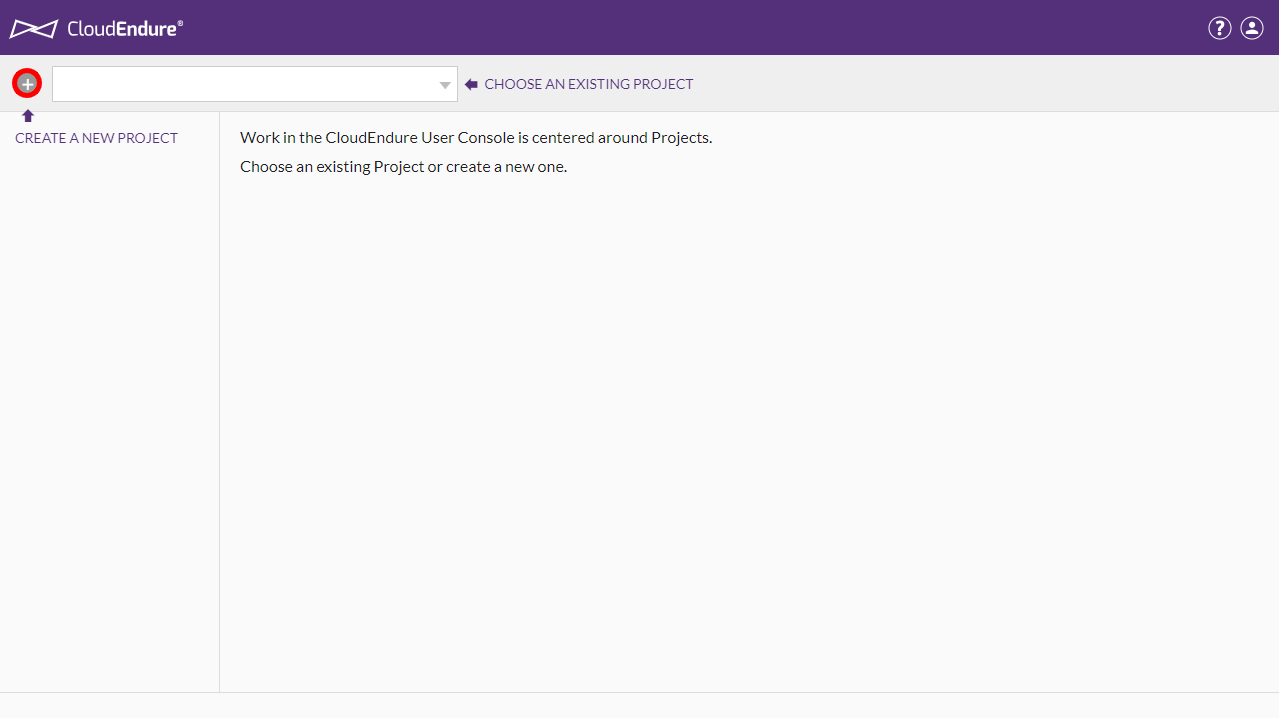The image prominently features a purple box at the top, containing a symbol resembling two tilted triangles with their top vertices touching, creating a bow-tie effect. The text "Cloud Endurer" is displayed, with "Endurer" in bold letters. To the right of this are two circles: one with a question mark and another with a generic profile picture. Below this section is a light gray area with a gray circle marked with a plus sign, encircled in red with a small arrow pointing at it. Adjacent is a text box offering a drop-down menu. To the right of the text box, a label reads "Choose an existing project," while below and to the left, another option states "Create a new project." Further to the right, the text explains the context: "Work in the Cloud Endurer user console, which is centered around projects. Choose an existing project or create a new one."